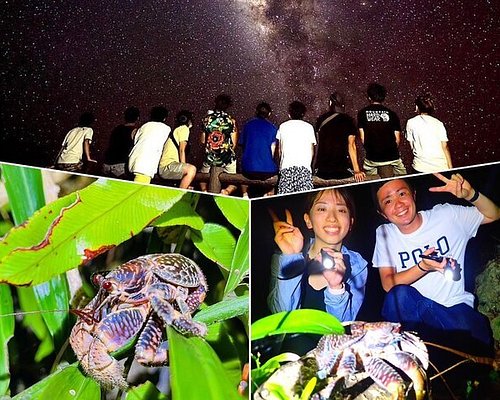This image collage, a rectangular montage wider than it is tall, artfully blends three distinct photographs. The top section captures a mesmerizing night scene where about ten people, with their backs turned towards the camera, sit on a horizontal wooden fence or log. They are stargazing under a stunning dark sky dotted with countless stars and illuminated by the Milky Way galaxy's ethereal glow.

The bottom right photo depicts a lively scene where a young woman on the left and a man on the right pose joyfully, both making peace signs and smiling at the camera under the night sky. They each hold a flashlight, illuminating a large land crab perched on a stump before them. The woman is dressed in a casual blue outfit, and the man pairs blue pants with a white t-shirt featuring a "Polo" logo.

In the bottom left photo, the focus shifts to a lush close-up of the land crab, emphasized by its intricate, segmented shells. The crab stands prominently on a leaf, surrounded by vibrant green foliage, showcasing the texture and uniqueness of this fascinating creature.

Combining elements of human connection, nature, and the celestial, this photograph collage tells a compelling story through its rich details and vivid imagery.